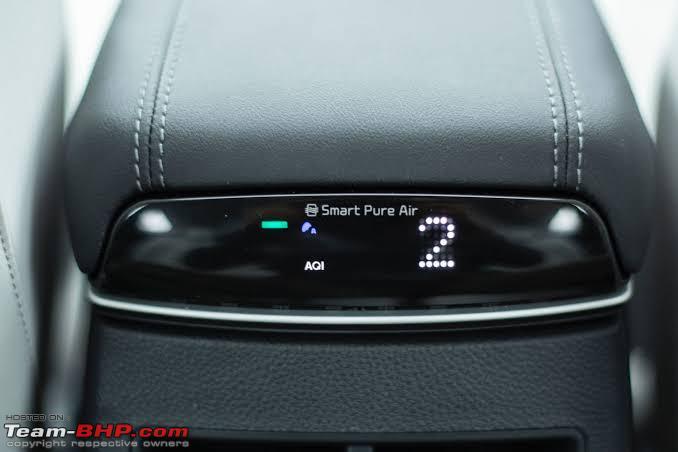The photograph depicts a black leather center console from a car, potentially from a luxury brand like Audi or Lexus. Dominating the central part of the console is a Smart Pure Air system embedded in the leather, with precise light gray stitching running along the edges. At the top of this console, the text "Smart Pure Air" is clearly visible, accompanied by the letters "AQI" (Air Quality Index) and a pixelated digital display showing the number "2" in white dots. This display area also features a small purple marking and the URL "TeamBHP.com" in bright red letters. The surrounding console area is a combination of gray and black leather materials, suggesting a sleek, high-end finish, akin to a dashboard or glove box of a car. Reflections and a green line can be seen in the display window of the air system, adding depth to the image. At the bottom left corner, the image bears the watermark "hosted on TeamBHP.com copyright respective owners."